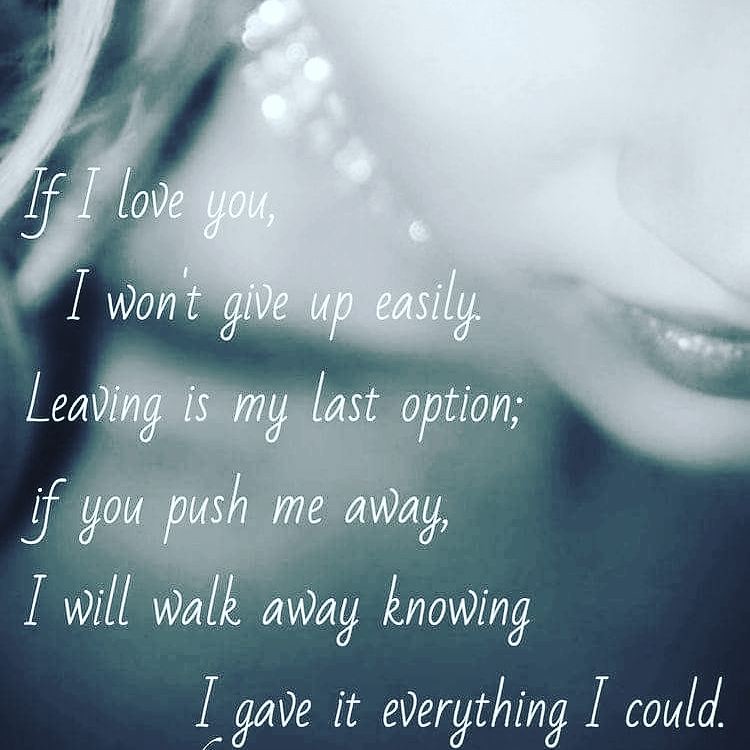The square image, reminiscent of a fashion magazine photo, features a close-up of a woman from the nose down against a light bluish background. The woman, possibly a model, has her blonde hair pulled back behind her ear, revealing a long neck adorned with a diamond necklace. Her lips are painted a striking red, and her expression appears serious. The photograph has a black and white tone, slightly faded, with bold white text that covers it. The text reads: "If I love you, I won't give up easily. Leaving is my last option. If you push me away, I will walk away knowing I gave it everything I could." The large lettering is prominently displayed across the image, emphasizing the poignant message.